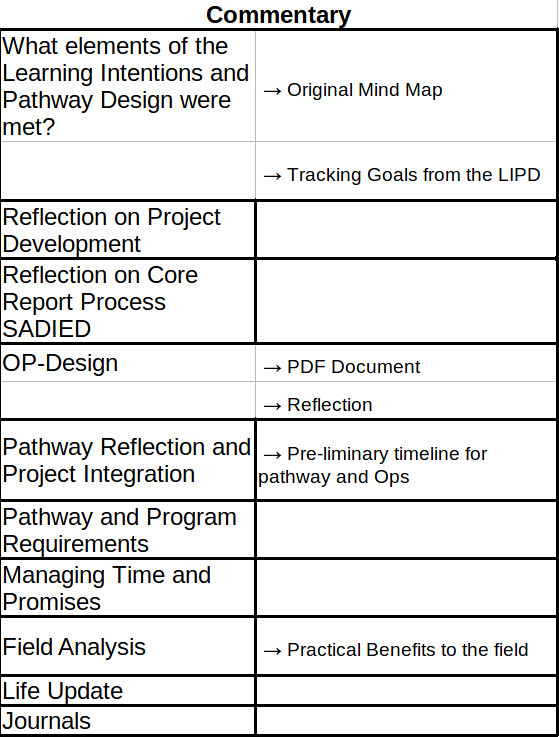The image depicts a detailed commentary section from a study. The page is structured with bold headers and is divided into two columns and 12 rows, separated by varying line thicknesses. The left column lists queries or categories related to learning intentions and pathway design, while the right column outlines the responses or related documents. From top to bottom, it includes: "What elements of the Learning Intentions and Pathway Design were met?" paired with "Original Mind Map"; "Tracking goals from the LIPD"; "Reflection on Project Development"; "Reflection on Core Report Process SADID"; "OP-Design", with an arrow pointing to "PDF Document"; "Reflection"; "Pathway Reflection and Project Integration", paired with "Preliminary Timeline for Pathway and Ops"; "Pathway and Program Requirements"; "Managing Time and Promises"; "Field Analysis", paired with "Practical Benefits to the Field"; "Life Update"; and "Journals". Some categories and responses remain blank or have directional arrows, suggesting further documentation is needed. The commentary systematically tracks goals, reflections, and essential components of the study's workflow.